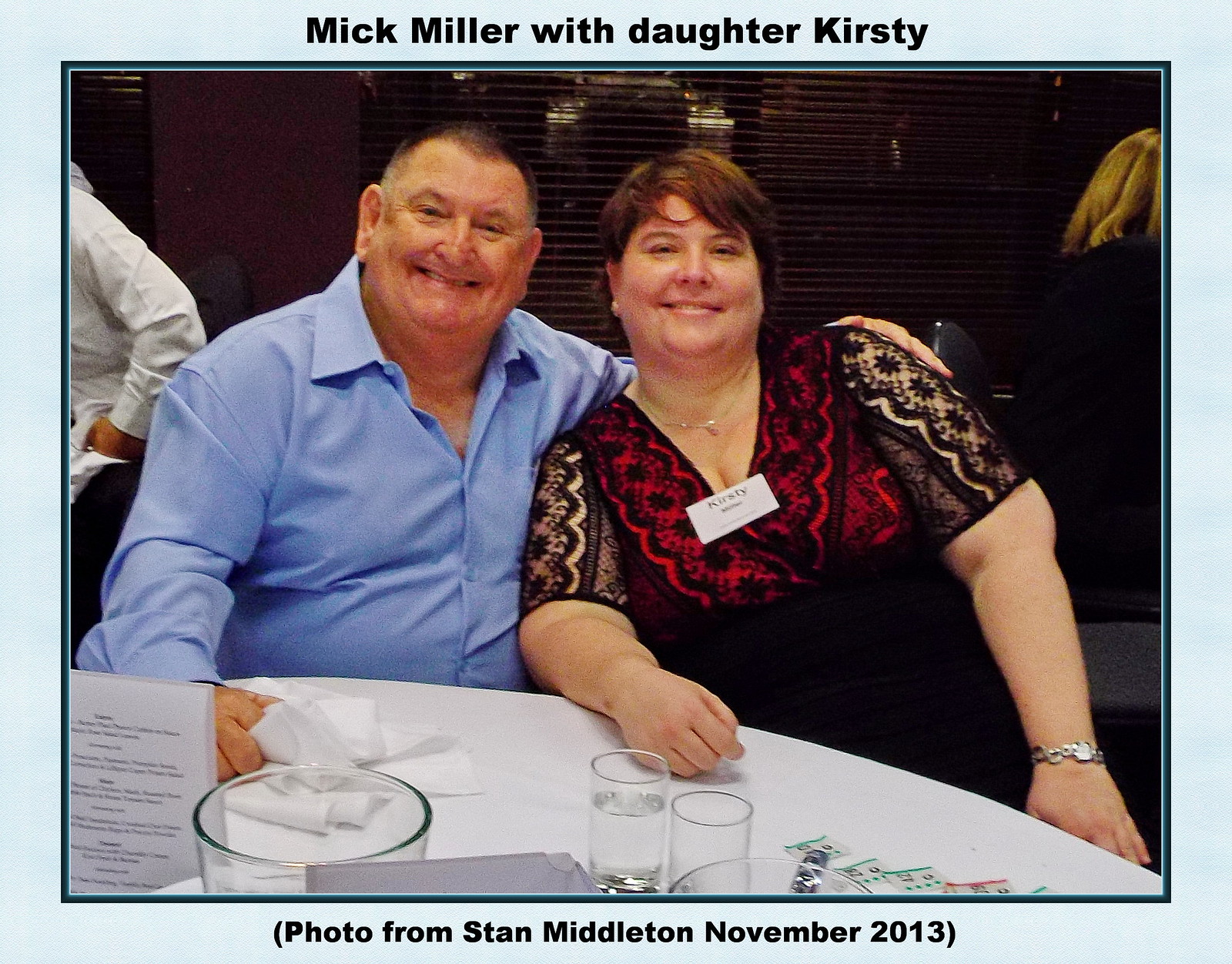The photograph, taken by Stan Middleton in November 2013, features Mick Miller and his daughter Kirstie seated at a round table, likely at a dinner event in an indoor setting. Mick, positioned on the left, is a slightly heavyset man in his early 60s, sporting a light blue button-down shirt with the top buttons undone, and a hint of graying black hair. He is smiling warmly and holding a napkin. Kirstie, seated on the right, appears to be in her 40s or 50s, with short brown hair and a name tag reading "Kirstie" clipped to her lacy black-and-red top. The setting has a restaurant-like ambiance with a window and blinds behind them, and a person in a white shirt partially visible to the left. On the table in front of them are several glasses and napkins, suggesting they may have just finished a meal. The image is bordered with a light blue frame, with the top bearing black text that reads "Mick Miller with daughter Kirstie" and the bottom reading "photo from Stan Middleton, November 2013."